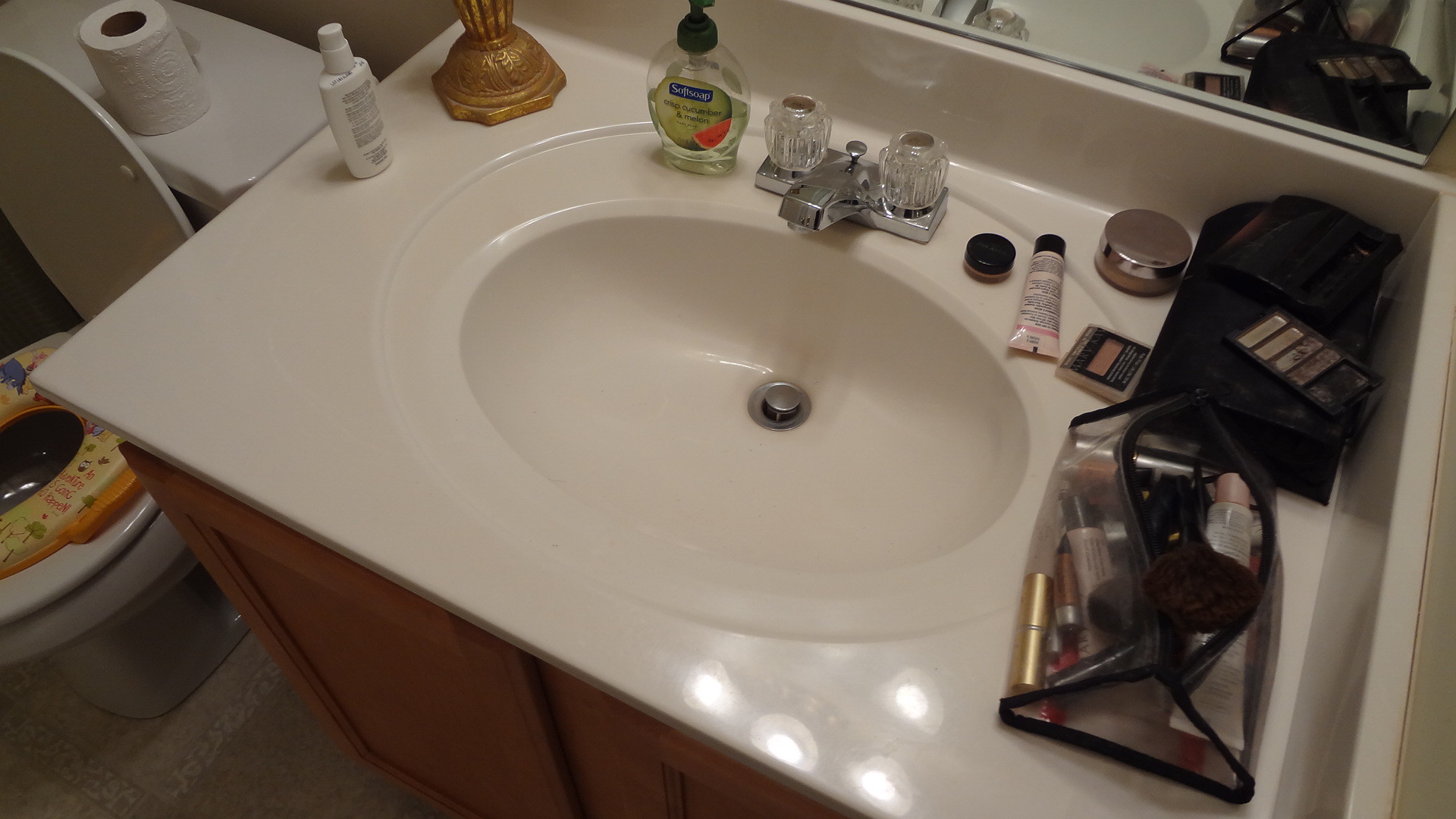This overhead photograph captures the details of a bathroom vanity nestled in the corner. The vanity itself is pristine white, featuring an integrated oval sink. The sink blends seamlessly with the white vanity top, while a silver faucet stands prominently. The faucet is equipped with clear, somewhat white plastic round knobs for hot and cold water control.

In the right corner of the vanity rests a black makeup bag, topped by a small black square item. Adjacent to this is an eyeshadow palette showcasing a range of brown shades. Positioned below this setup, a clear plastic makeup bag with black edges reveals various makeup items inside.

Moving leftward, a round, short jar with a silver lid is accompanied by a multi-colored square container—black on top, brown on the side, and featuring a reddish rectangle. Next to this, a small white tube with a brown cap lies. Further left, a round black container sits near these items.

On the left side of the faucet, a jar of soft soap with a pump top is visible. Just below this area, the base of a gold-colored object can be seen, leading to a small white plastic jar with a pump, rectangular in shape.

The scene extends to the left where the top of the toilet tank is visible, supporting a roll of white toilet paper. The toilet seat is raised, making way for a child’s potty seat that is yellow and orange around the edge. The array of personal items and toiletries provides an intimate glimpse into a daily routine space, meticulously organized with everyday essentials.